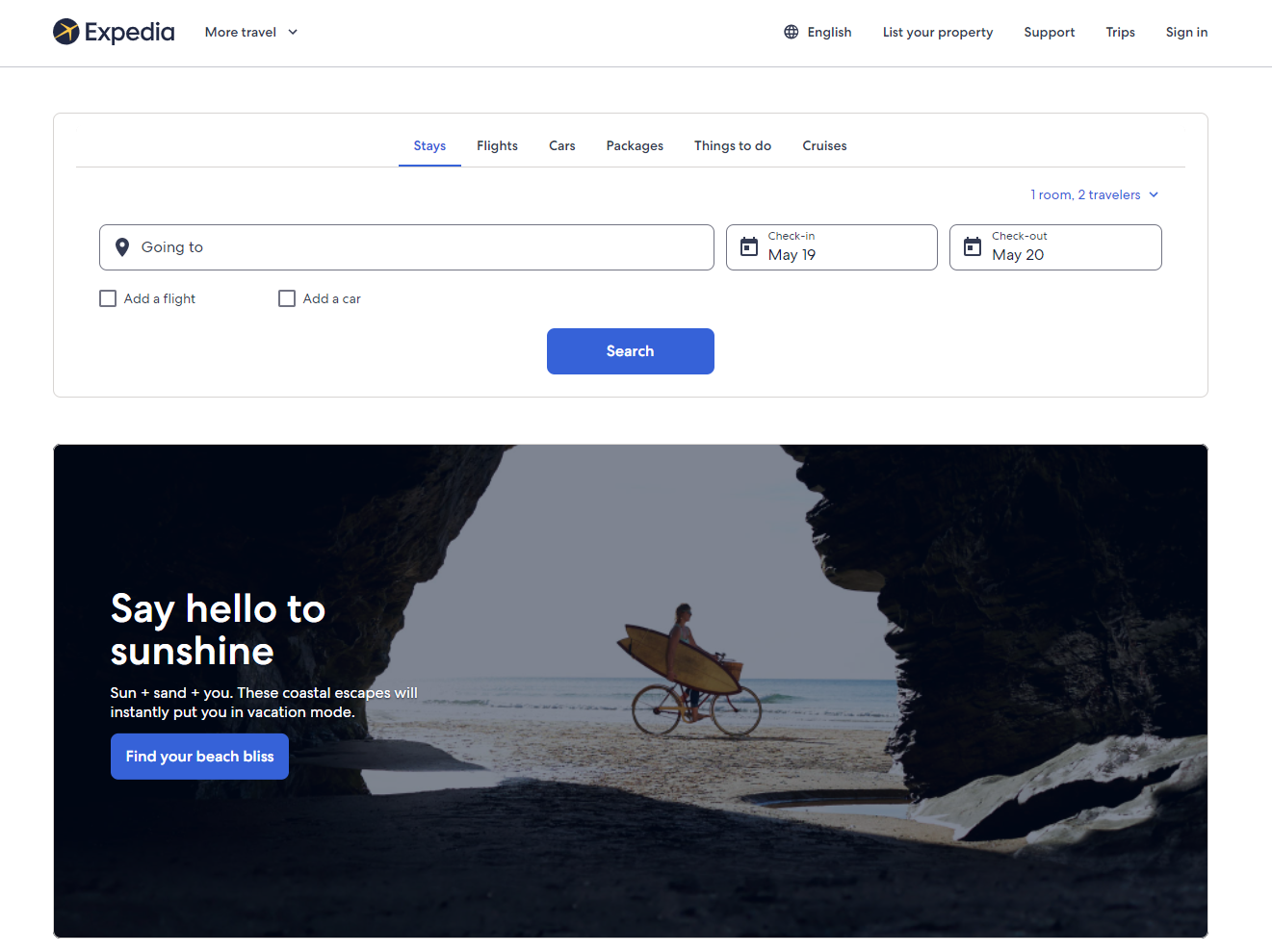This is a detailed caption for an image of a screenshot from the Expedia website:

The image showcases a screenshot of the Expedia website, featuring a clean and modern design. In the top left corner, there's the recognizable Expedia logo followed by the word "Expedia." Adjacent to that is a link labeled "More Travel." Moving to the top right corner, the navigation options include "English," "List your property," "Support," "Trips," and "Sign In," all against a white background.

Directly below this header is a navigation bar with categories: "Stays," "Flights," "Cars," "Packages," "Things to Do," and "Cruises." Beneath this bar is a search tool that initiates with a map pin icon labeled "Going to," followed by fields for "Check-in" on May 19th and "Check-out" on May 20th, complete with calendar icons for date selection. A prominent blue search button with the word "Search" written in white letters is centrally located for easy access.

Below this search functionality, an evocative image captures attention. The image is framed with black borders on the left, right, and bottom. At the heart of the image, a person rides a bicycle while expertly balancing a surfboard. The scene is set on a beach, with the vast ocean and a clear blue sky contributing to the serene atmosphere. Superimposed text over the image reads "Say hello to sunshine" on the left. Beneath the image, promotional text declares, "Sun + Sand + You. The coastal escape will instantly put you in vacation mode." An inviting blue button with "Find your beach" written in white letters encourages users to explore further.